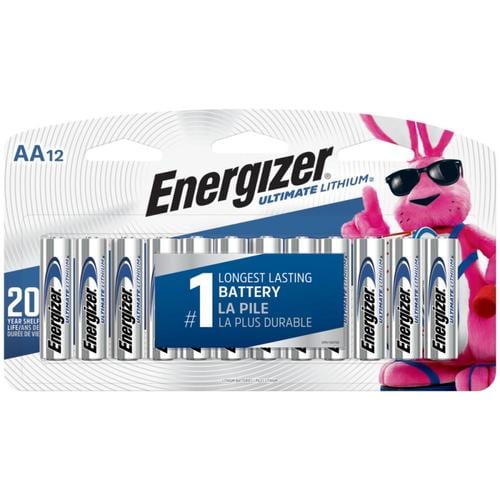The image depicts a package of Energizer AA batteries, designed for retail display with a distinctive rounded top resembling an arch, diverging from the more common square packaging. The package prominently states "12," indicating it contains 12 batteries. The brand "Energizer" is displayed diagonally from the southwest to the northeast. The package advertises "Ultimate Lithium" batteries and features the iconic Energizer Bunny, wearing sunglasses and holding up his right hand with a "#1" gesture, positioned on the right side of the packaging. The batteries are enclosed in a bubble pack, and above them, the text "Number 1 Longest Lasting Battery" is highlighted, emphasizing the product's durability. There is also a partially obscured "20" on the left side, further hinting at some performance metric. These are identified as "LAPOW" batteries, noted for their superior longevity.